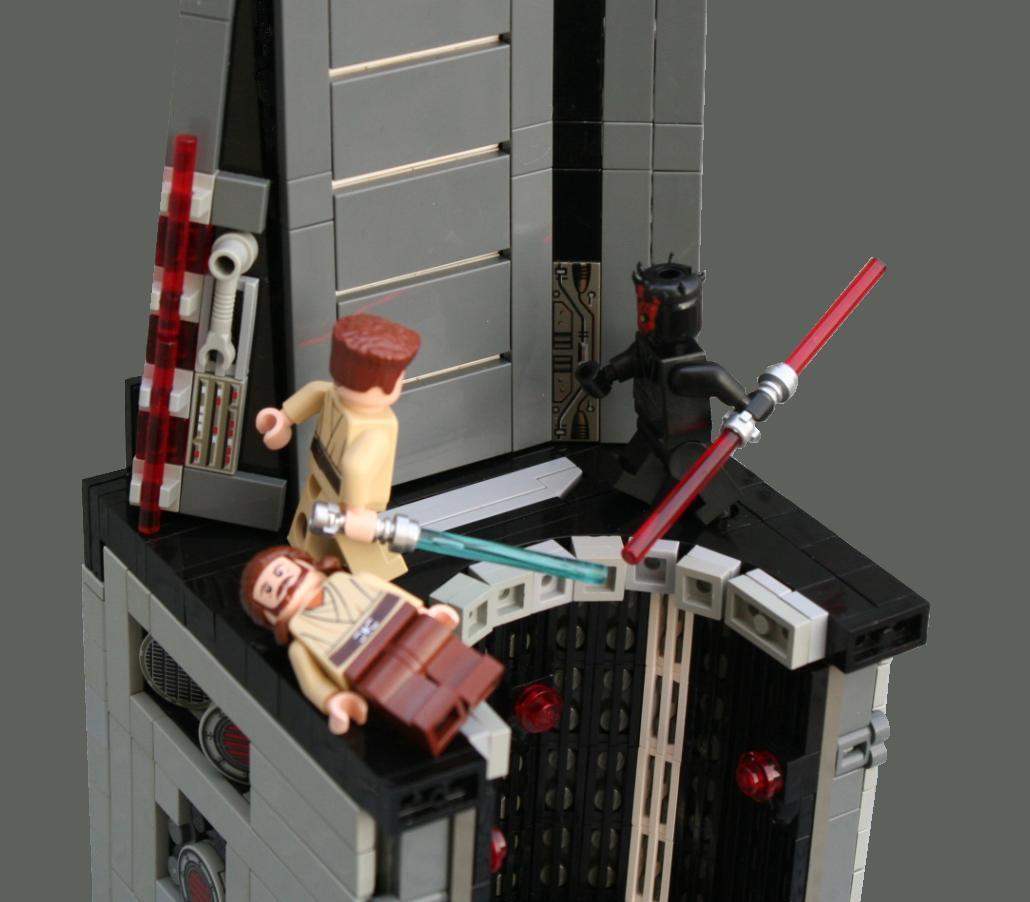The image captures an elaborate Lego recreation of a pivotal scene from Star Wars Episode I, where Qui-Gon Jinn faces off against Darth Maul while Obi-Wan Kenobi rushes to intervene. Central to the scene is a tall, gray tower constructed from small, meticulous Lego blocks. The tower stands beside a black platform, which features a circular cutout leading into a deep pit, reminiscent of the Theed Generator Complex. On the platform lie three Lego figurines, positioned to mirror the dramatic moment. 

To the left, the Lego figure of Qui-Gon Jinn lies on the ground, distinguished by his light brown top, dark brown legs, and detailed cylinder head adorned with a painted beard and long brown hair. Nearby, the figure of Obi-Wan Kenobi stands with his back turned, clutching a blue lightsaber with a silver hilt in his right hand. Opposing him across the platform is Darth Maul, recognizable by his black and red face, black spiked hair, and a menacing double-sided red lightsaber. The figures are encircled by further light gray panels and Lego pieces meticulously scattered to provide context, all set against a neutral gray background that emphasizes the central action of this iconic Star Wars duel.